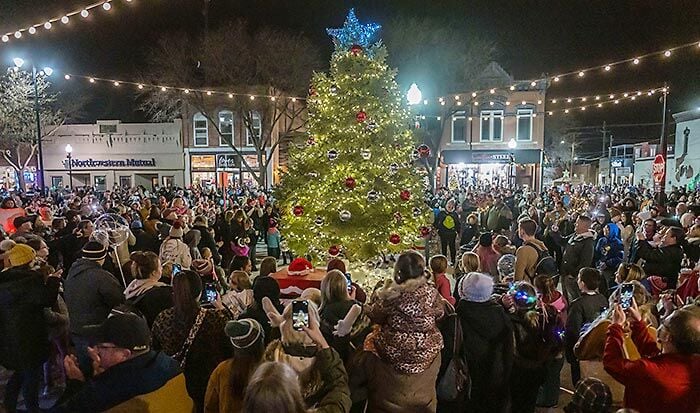This vividly detailed photo captures a festive Christmas tree lighting ceremony in a quintessential small-town American square. Centered in the scene is a beautifully lit Christmas tree adorned with red, silver, and blue ornaments, crowned with a prominent blue star. The tree is enveloped by an enthusiastic crowd of over a hundred people of all ages, many of whom are taking photos with their smartphones. The crowd, thick and densely packed, includes children perched on parents' shoulders and individuals donning winter attire such as knitted hats, jackets, and gloves. The surrounding atmosphere buzzes with joy and warmth, amplified by string lights that crisscross overhead, casting a magical glow over the town square. In the background, a mix of two-story shops and buildings, including a distinctly labeled Northwestern Mutual building, creates a picturesque backdrop. A stop sign stands vividly to the right, adding a familiar touch of small-town America. The scene is richly festive, embodying the spirit of Christmas in a close-knit community.